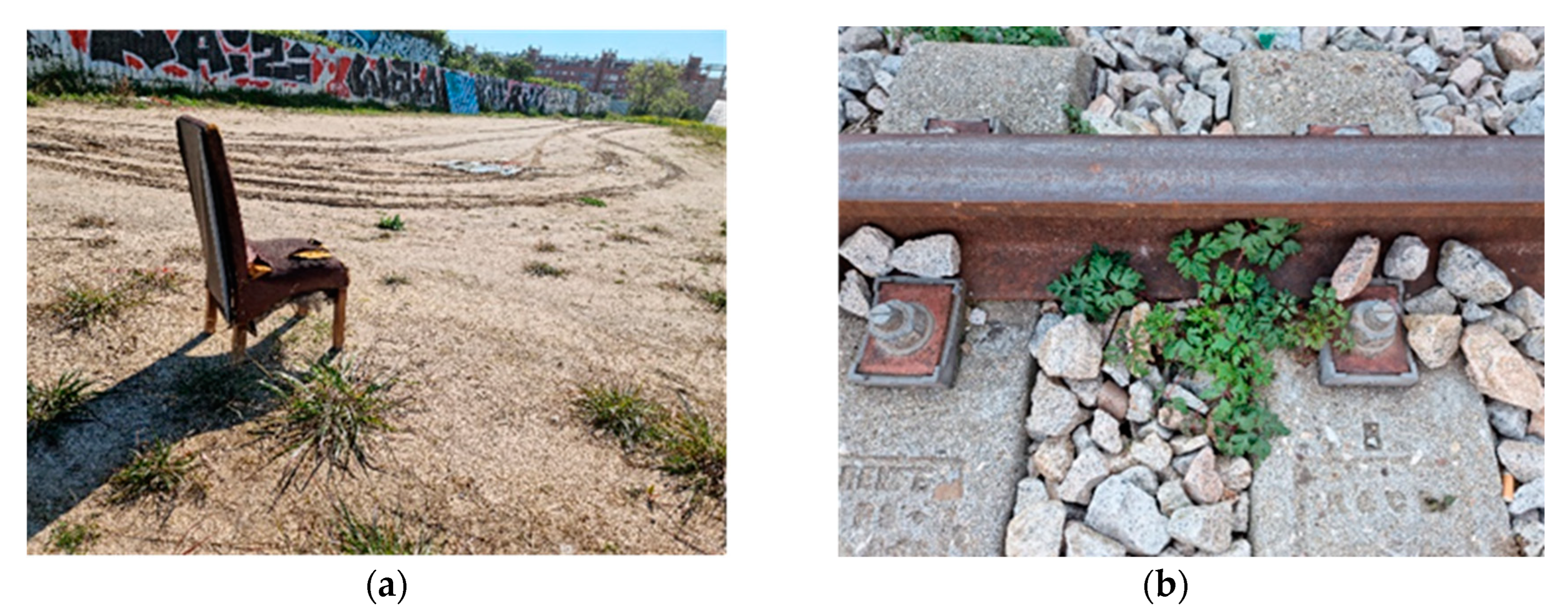The composite image set presents two distinct scenes, labeled A and B. 

The left image, labeled A, captures a wide-angle view of a desolate, sandy area punctuated by sparse grassy shrubs and tire tracks imprinted on the ground. Dominating the foreground is a dilapidated, empty chair with a brown back and a broken seat pad. Shadowed to its left, the chair appears very old and torn. The background reveals a wall adorned with vibrant graffiti, prominently featuring the text “NAI2” in black lettering against a red background. The scene unfolds under daylight, casting a raw and gritty atmosphere over the abandoned chair and its surroundings.

The right image, labeled B, provides a close-up view of a horizontal train track. The track itself is a large piece of iron, its surface mottled with rust, transitioning from a deeper brown to more orange hues along the sides. Bolts secure the track into a foundation of assorted gravel stones in shades of grey, beige, and orange. From beneath the track, green foliage and small plants sporadically sprout, highlighting the encroachment of nature upon the man-made structure. Concrete supports can be seen extending under the rail on both sides, supporting the rusted track above.

Overall, the set juxtaposes an expansive, barren landscape with a detailed, confined segment of railway, each image characterized by elements of decay and encroachment by nature.